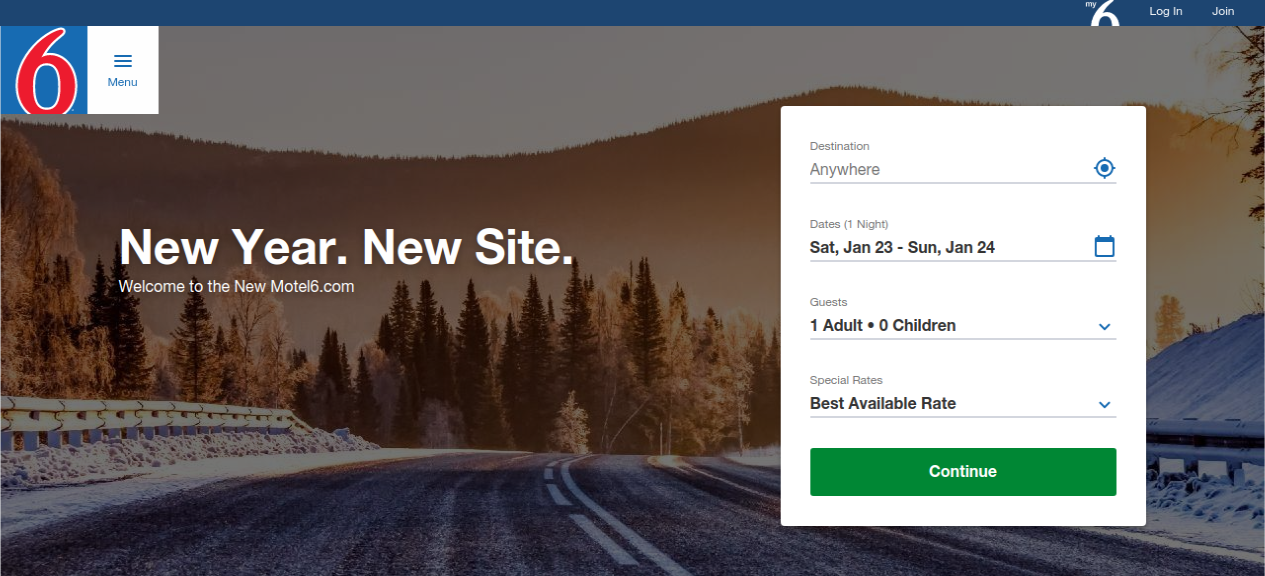The image depicts a website interface for a company named Motel 6. At the top of the screen, a horizontally oriented, navy blue bar stretches across, featuring the options "Login" and "Join" on the right side, accompanied by the ASICS logo. Below this blue bar, another company logo is displayed - a square with a blue background and the word ASICS in red text. 

To the left of this logo, there is a menu button which, when clicked, expands to show additional navigational options. On the right side of the screen, there is a floating white box labeled "Destination," where users can input their desired travel location. This box also includes fields for "Dates," allowing users to specify their stay period, as well as options for indicating the number of guests and the desired rate. Below these input fields, a green "Continue" button is available for users to proceed once all information has been entered.

The background of the screen is adorned with a scenic photo featuring mountains, trees, and a snowy road. Overlaying this backdrop are the words in white text: "New Year, New Site. Welcome to the newmotel6.com."